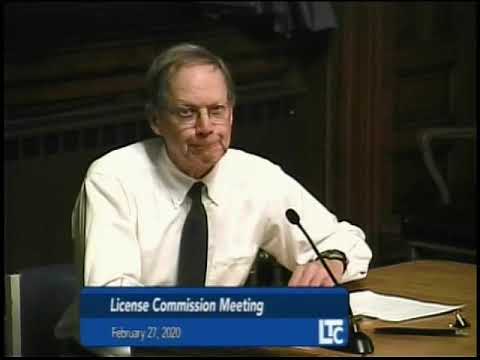The image captures a televised city council or License Commission Meeting dated February 27, 2020. Central in the frame is an older Caucasian gentleman, approximately between 60 to 65 years old, with grayish-brown hair styled in a side comb over, and wearing square glasses. The man, who has a pale peach complexion, is dressed in a white button-down shirt paired with a dark tie. He is seated at a light-colored wooden table, positioned slightly off-center to the left. On the table is a white piece of paper and a black microphone, directed towards his mouth. The text overlay at the bottom of the image includes a blue lower third text box reading "License Commission Meeting" in white letters, accompanied by the date February 27, 2020, against a light blue background. The LTC logo is also present in the bottom right corner. The overall ambiance is professional, although the man appears to have an unpleasant smirk or scowl on his face, possibly directed at someone off-camera. The background lacks other people, indicating the meeting might be sparsely attended.